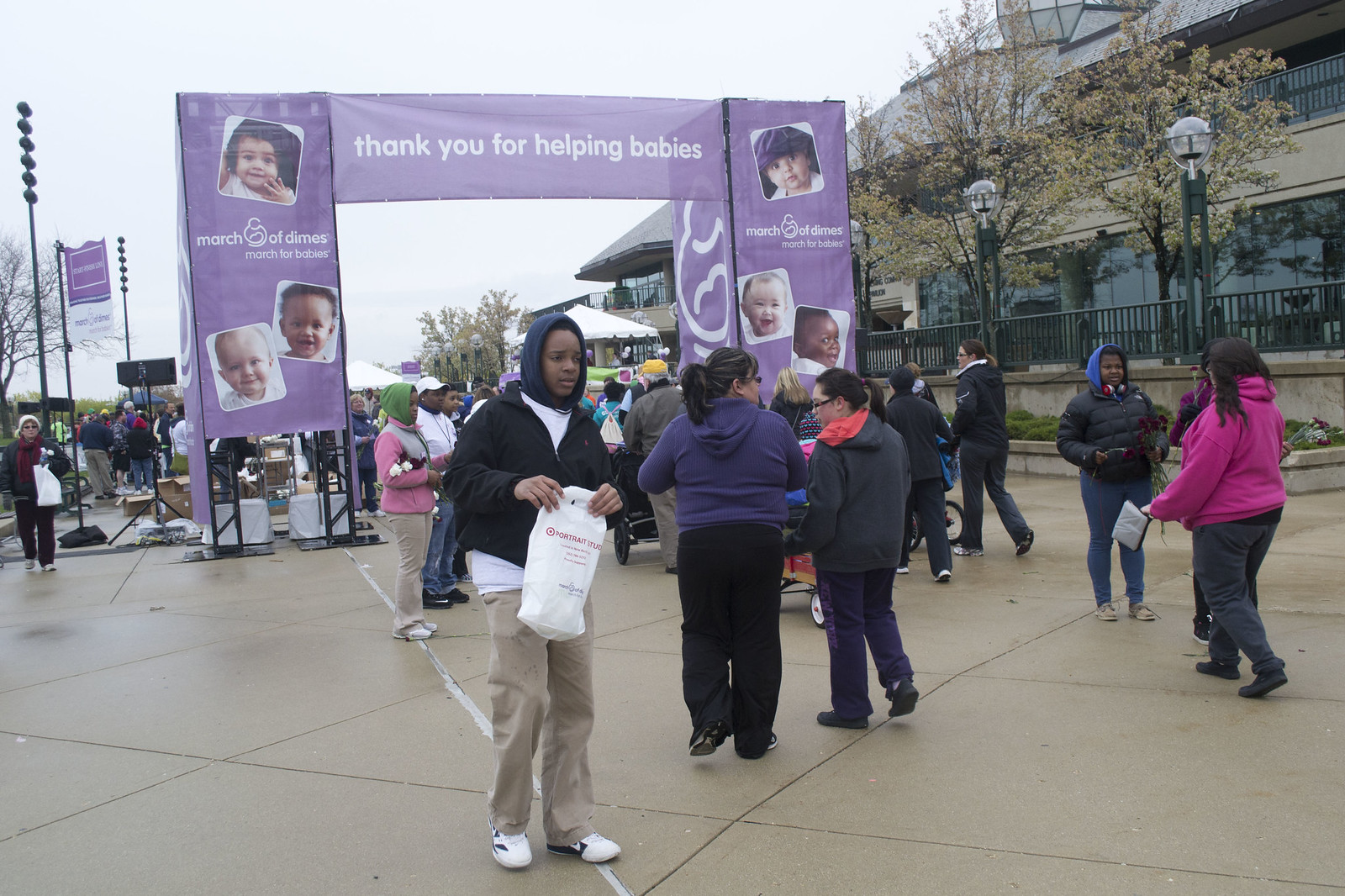The photograph depicts a bustling outdoor event on a cement or asphalt pathway with numerous people either walking or standing around. Dominating the center of the image is a gateway-like arch structure adorned with two large vertical banners in purple, each featuring three pictures of babies and white writing beneath them. Joining these banners at the top is a horizontal banner reading "Thank you for helping babies," suggesting the scene is part of a charity event, likely a "March of Dimes" or "March for Babies." To the right of the archway stands a multi-story building with extensive glass windows, three lampposts, and a green railing. Trees dot the scene, adding a touch of greenery. Various colors, including brown, gray, white, red, pink, purple, blue, orange, and light green, are present throughout the image, creating a vibrant, community-focused atmosphere under a white sky. Notably, a man wearing a hooded jacket and holding a white bag is seen walking towards the archway, adding a human element to the lively gathering.